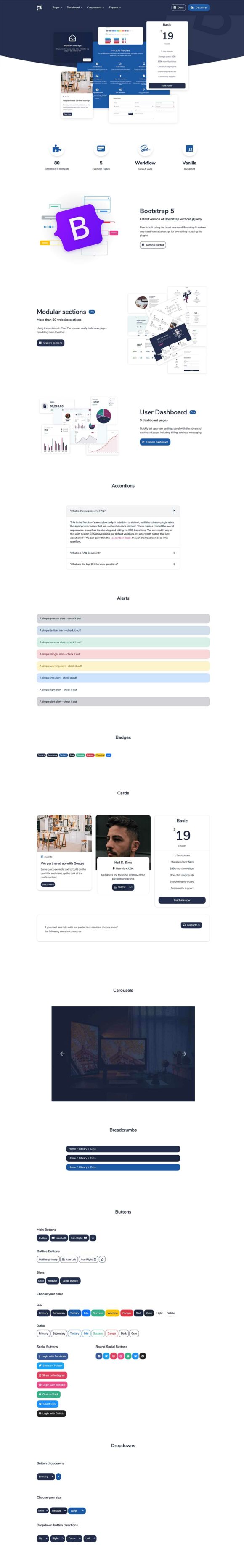The image depicts a multi-page layout of a website, albeit difficult to discern in its entirety. One prominent feature on the first page is a purple box with the letter "B" inscribed on it. This purple box appears to have arrows on both the left and right sides, creating a 3D effect as if it is protruding from the screen. Additionally, the page contains labels such as "Bootstrap 5," "User Dashboard," and "Modular Sections." It also includes graphical elements, specifically a bar graph with fluctuating values, though the specific data points and text on the graph are not easily legible. The overall theme seems to be centered around web development and user interface design.